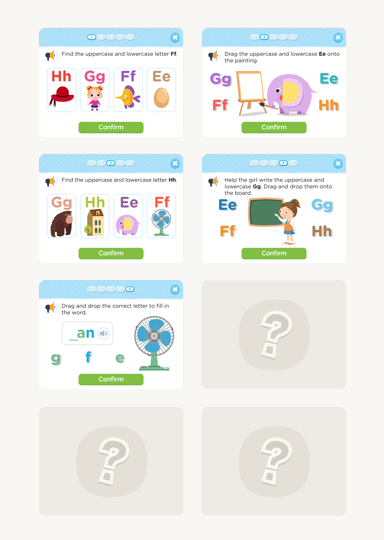Here is a cleaned-up and detailed description of the caption:

---

The screenshot features a children's app with a tan-cream colored background. There are four primary interactive tiles arranged in two rows of two, totaling eight tiles. The bottom two tiles and the second tile from the bottom right display question marks. 

Each of the other tiles has a light blue top banner and a white background. This app appears to be focused on teaching the alphabet. 

1. **Top Left Tile:** Displays the sequence "H H G G F F E E" with corresponding icons below and a green 'confirm' button at the bottom.
   
2. **Top Right Tile:** Contains instructions that read "Drag the uppercase and lowercase E onto the painting G G F F E E H H" followed by a green 'confirm' button.

3. **Bottom Left Tile:** Similar to the top left tile but with the letters arranged differently and different icons, also featuring a green 'confirm' button.

4. **Bottom Middle Tile:** Describes an alphabet-related activity with the typical green 'confirm' button.

This setup outlines an interactive and engaging approach for children to learn the alphabet, emphasizing various activities and confirmatory actions.

---